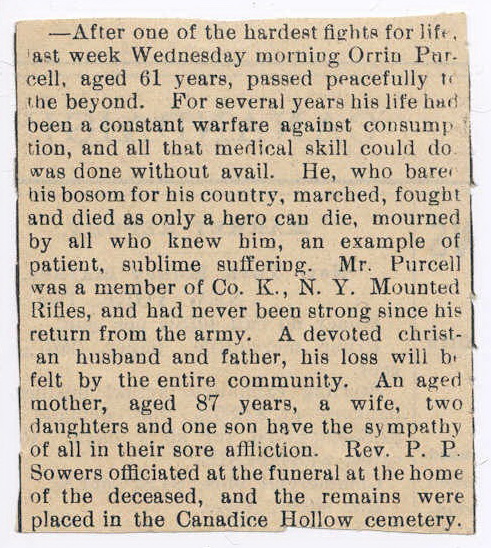The image shows a detailed obituary for Oren Purcell, aged 61, who peacefully passed away on a Wednesday morning after a prolonged battle with consumption. The obituary highlights his heroic service as a member of Company K in the New York Mounted Rifles during the war, noting that his health had never fully recovered since returning from the Army. It lauds him as a devoted Christian husband and father, whose passing deeply affects his community. He is mourned by an aged mother, 87, his wife, two daughters, and one son. Reverend P.P. Sowers conducted the funeral service at Mr. Purcell's home, and he was laid to rest in Canada's Hollow Cemetery. The obituary reflects on his life of patient and sublime suffering and honors his courageous contributions both in life and in service to his country.